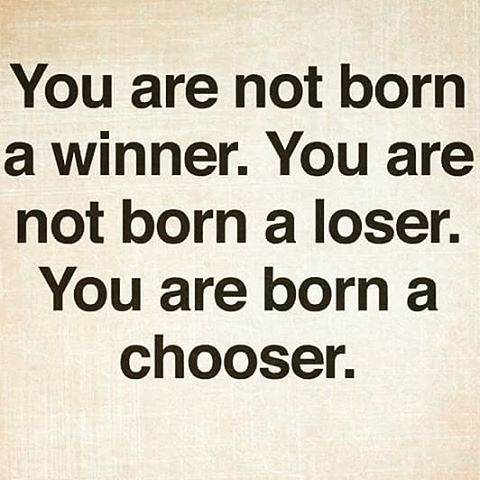The image is a motivational poster with a white background and black bold letters. It features three straightforward sentences, each on a separate line, reading: "You are not born a winner. You are not born a loser. You are born a chooser." The text is clear and well-punctuated, providing an impactful message. Although primarily white, the background has subtle variations in shading, with darker areas visible in the upper left and lower right corners. This poster, reminiscent of a motivational billboard or an Instagram post, serves as a simple yet powerful reminder of personal agency and choice in life.